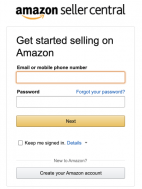The image is a screenshot of the Amazon Seller Central login page. At the top, the Amazon logo is prominently displayed, featuring the characteristic yellow "swoosh" arrow under the word "Amazon." Below the logo, the text reads, "Get started selling on Amazon."

Centered on the page is a white input box outlined in yellow, prompting the user to enter their email or valid phone number, with the field itself currently blank. Directly below this input field, there is a space for entering a password. Adjacent to the password field on the right side is a blue "Forgot your password?" link, allowing users to recover their password if needed.

Further down, there is a yellow rectangular button labeled "Next," which enables users to proceed with their login. Near the bottom of the page, a gray checkbox is available for users to select the "Keep me signed in" option, accompanied by a blue "Details" link for more information about this feature.

Finally, at the bottom of the image, the text "New to Amazon?" appears in gray, followed by another prompt, "Create your Amazon account," encouraging new users to sign up.